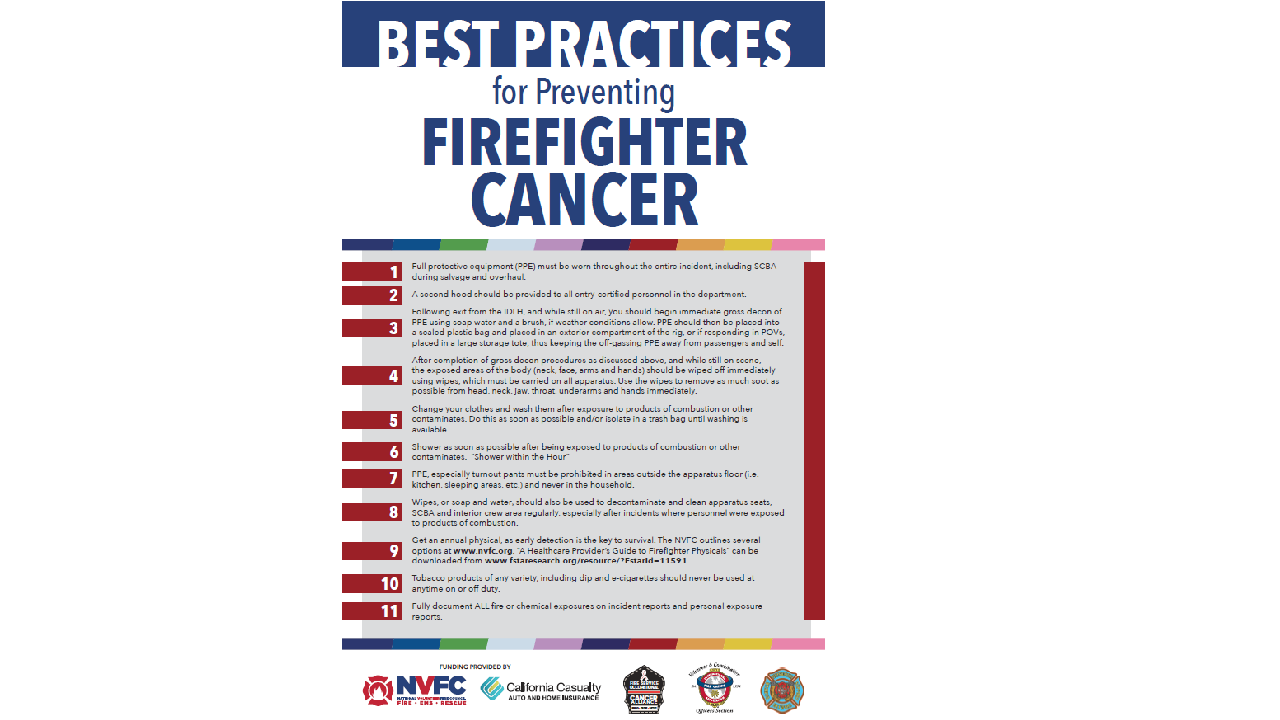The poster is an informational health guide on a white background, emphasizing cancer prevention for firefighters. At the very top, a dark blue banner with bold white lettering reads "Best Practices," followed by "For Preventing" in dark blue lettering on a white background, and "Firefighter Cancer" also in dark blue. Beneath this is a multi-colored line transitioning through various hues including black, blue, green, light blue, light purple, bright red, light yellow, and pink. This line separates the top section from a gray area containing 11 small, illegible sentences, each numbered 1 through 11 next to a red bar. The red bar also runs vertically down the right-hand side of the poster. At the bottom, a similar multi-colored line spans from left to right, above which are five logos. Two logos are legible, reading "NVFC" in red and blue, and "California Casualty" in blue with black text. Three other logos are present but illegible. The poster's main focus is on various practices for cancer prevention among firefighters, including the usage and cleaning of Personal Protective Equipment (PPE) and SCBA, as indicated, though specific text details are too small to read.